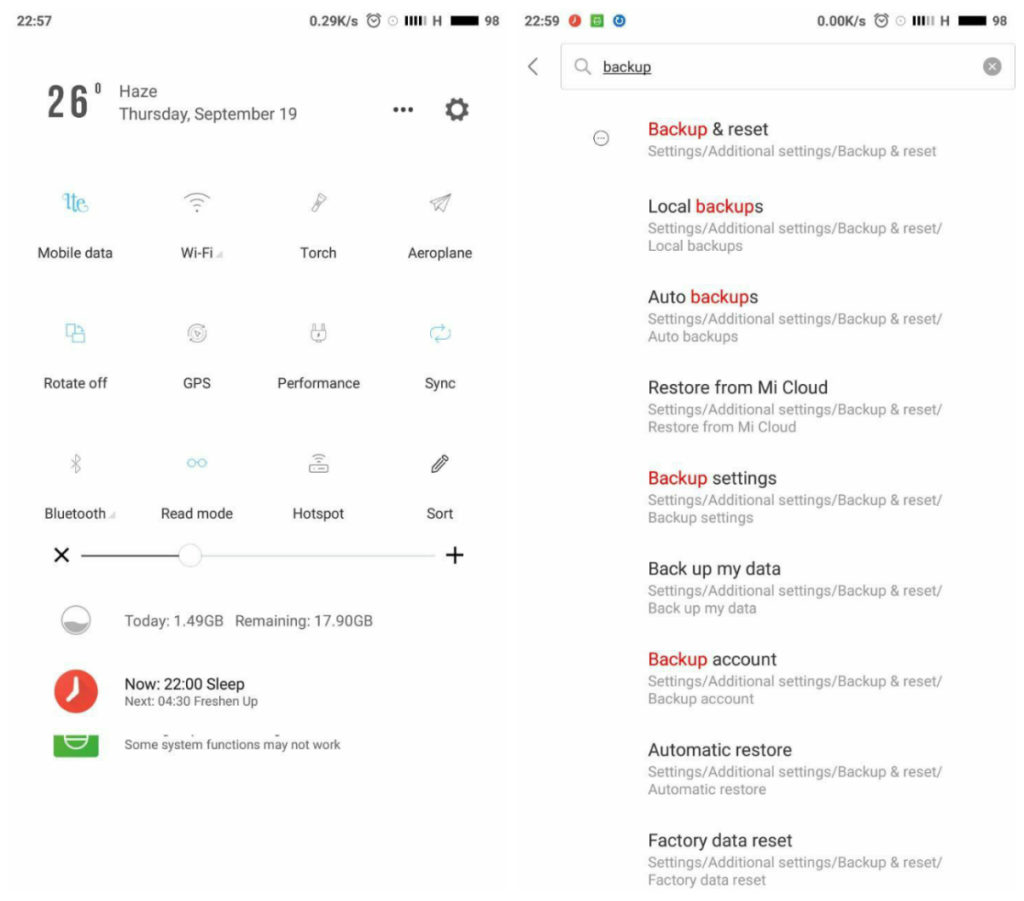In the image, the interface of a mobile device is displayed. At the top right, there is a search bar with the term "backup" highlighted in red, while other terms are black. 

Below the search bar, search results are listed as follows:
1. "Backup and reset" under "Settings > Additional settings > Backup and reset."
2. "Local backups" under "Settings > Additional settings > Backup and reset > Local backups."
3. "Auto backups" following the same path ending with "Auto backup."
4. "Restore from Mi Cloud" under "Settings > Additional settings > Backup and reset > Restore from Mi Cloud."
5. "Backup settings" under which several subsections appear, including:
    - "Backup my data"
    - "Backup account"
    - "Automatic restore"
    - "Factory data reset."

On the left side of the interface, there is an icon or menu option. At the top left corner, information about the current weather is shown: "26 degrees, haze." The date is indicated as "September 19." 

A settings icon is located on the top right within the notification panel. The panel shows different toggles for functionalities:
- Mobile data: on (blue)
- Wi-Fi: off
- Torch: off
- Hello Brain: off
- Rotate: on (blue)
- GPS, Performance, and Sync: on (blue)
- Bluetooth and Red mode: on (blue)
- Hotspot: short form shown

Additionally, there is a brightness bar positioned in the center of the notification pane. 

At the bottom of the screen:
- Data usage information "Today: 1.49 GB used, remaining 17.7 GB of 17.9 GB."
- Current time indication "22:00."
- Sleep mode indication
- Options "Next" and "Off"
- Rotate suggestion
- Refreshing app notification
- A red alarm clock icon on the left side

A message at the bottom states, "Some system functions may not work," accompanied by a small green icon on the left.